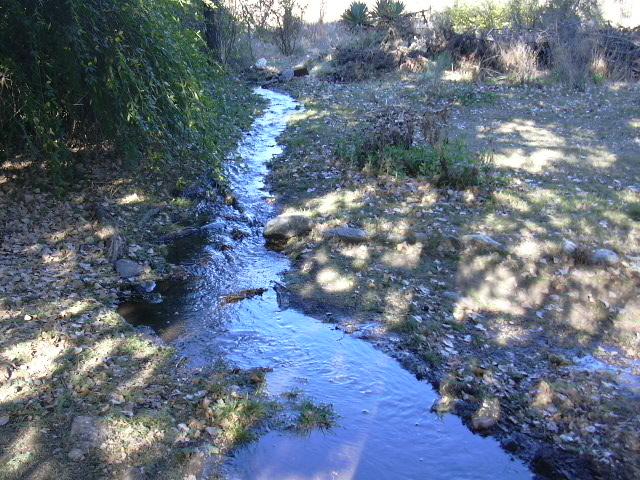A picturesque forest scene bathed in sunlight, with dappled shadows suggesting it's a bright day. At the center, a small blue stream meanders from the bottom right towards the left, flanked by lush greenery and rocky banks. The foreground features abundant grass blending into bushels of leafy bushes, interspersed with a mix of pebbles and gravel. A solid ground on the stream's opposite side appears easily crossable, enhancing the sense of accessibility. Towering trees, possibly including a weeping willow, cast gentle shadows, and drooping branches frame the top left of the image. Rich vegetation, including more green bushes and patches of sunlight filtering through the canopy, underscores the natural beauty of this serene forest setting.